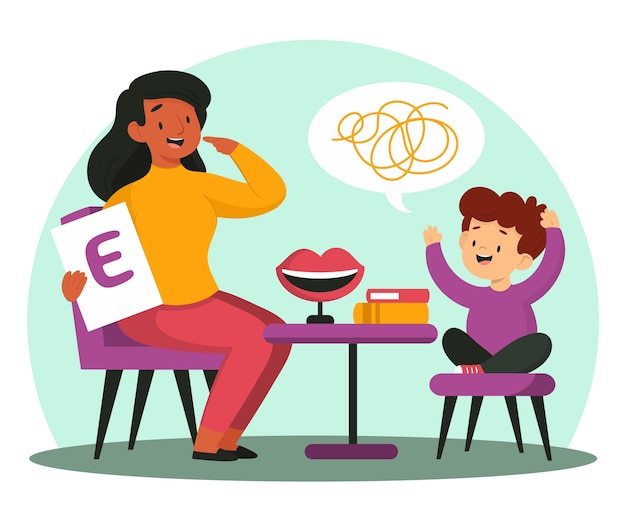In this animated illustration, an adult woman and a young boy are seated across from each other at a low, purple table with a single black rod and black leg in the center, a purple base, and a noticeable shadow underneath, creating a circular effect. The woman, with tan skin and black hair, is wearing a long-sleeved yellow (or golden orange) top and pink (or red) leggings. She sits on a purple chair with black legs and holds up a piece of white paper displaying a bold, purple letter "E." The young boy, who has light skin and reddish-brown hair, sports a long-sleeved purple shirt, black pants, and red sneakers. He sits crisscross on a smaller, purple stool with black legs, mumbling or talking, as indicated by a speech bubble filled with tangled yellow scribbles. On the table beside them is a large sculpture-like object of a mouth with red lips, smiling, mounted on a base. Also present on the table are two stacked books: a golden book at the bottom and a red book on top.